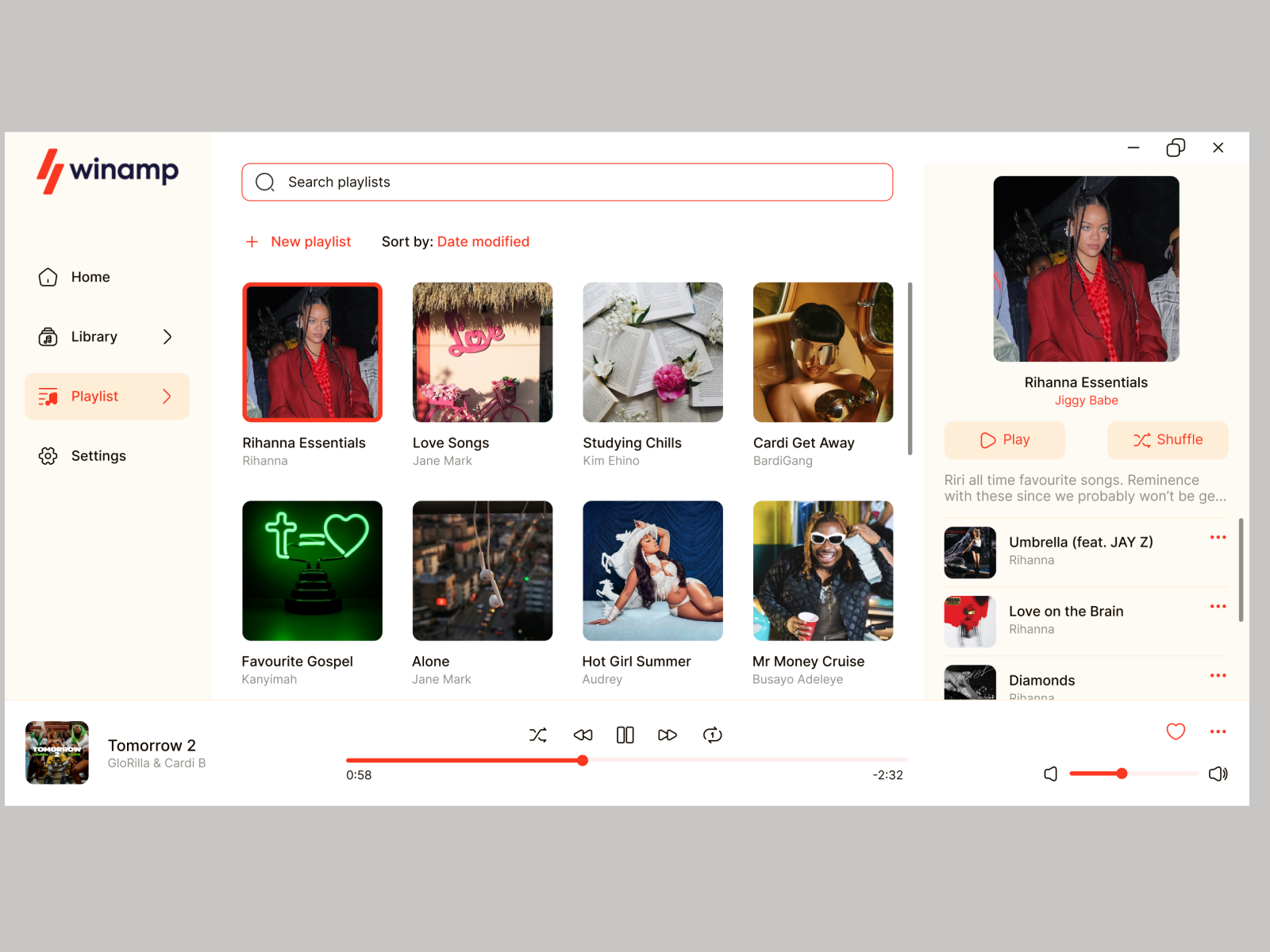The image is a detailed screenshot of the Winamp music player application, displayed against a dark gray background, highlighting a white central interface area. In the top left corner of the interface, there's the recognizable Winamp logo, featuring the word "Winamp" in black text adjacent to a stylized red icon.

Directly below the logo, a vertical navigation bar provides access to various sections of the website, listing four options: Home, Library, Playlist, and Settings. The "Playlist" option is prominently marked with a yellow background and red text, indicating it is the currently active section.

The central area of the interface displays several user-generated playlists, including names like "Rihanna Essentials," "Studying Chills," "Alone," and "Mr. Money Cruise." Each playlist title acts as a clickable link to access the respective music collection, with "Rihanna Essentials" highlighted by a red border, signifying it is the currently selected or playing playlist.

On the right side of the interface, a vertical box titled "Rihanna Essentials" reveals a detailed list of songs within the playlist. Each song listing is accompanied by "Play" and "Shuffle" buttons for on-the-fly playback options.

At the bottom center of the image, a horizontal control bar showcases the current song being played. This bar is equipped with standard media player buttons, including pause, fast-forward, and replay functionalities. Additionally, the bottom right section contains a volume adjustment bar, allowing users to fine-tune the audio output.

Overall, the screenshot encapsulates the user-friendly layout and interactive features of the Winamp music player application.